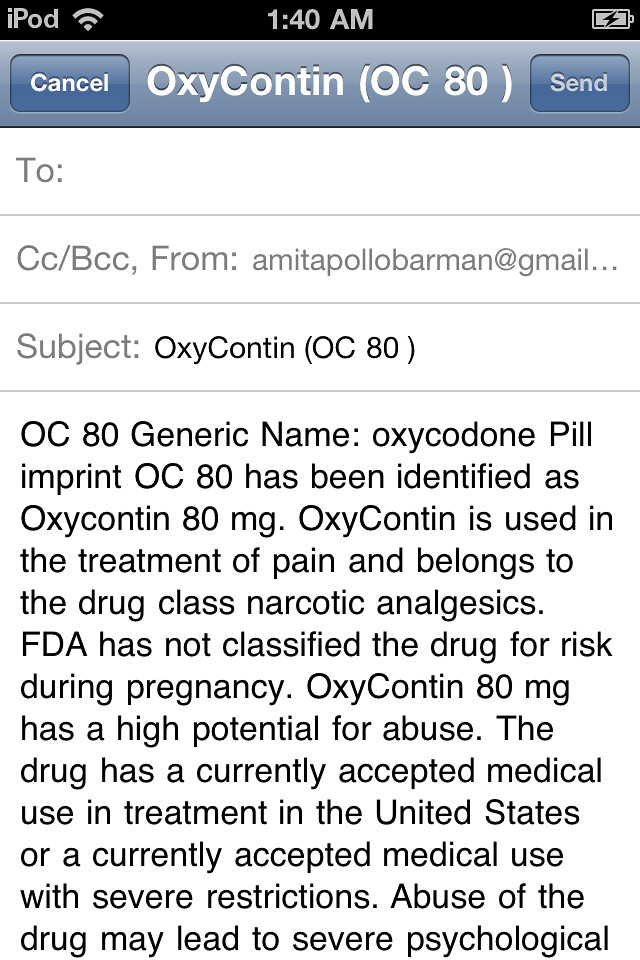The image shows a detailed screenshot of an email draft on an iPod. At the top of the screen, the iPod's time reads 1:40 AM, accompanied by the Wi-Fi signal, and the battery status indicates it is charging. Below this, a banner displays the options "Cancel" and "Send." The "To," "From," and "Subject" fields are laid out in horizontal lines. The "From" field contains the sender's email address, amitapolobaman@gmail.com, and the "Subject" field is titled "OxyContin OC80." The body of the email begins with "OC80 generic name, oxycodone," explaining that the pill imprint OC80 is identified as OxyContin 80mg. The text further outlines that OxyContin is utilized in pain treatment and is classified under narcotic analgesics. It mentions that the FDA has not classified the drug for pregnancy risk and notes the drug's high potential for abuse despite its accepted medical use in the United States under severe restrictions. The email discusses the severe psychological risks associated with drug abuse. The overall setting suggests someone is composing an email about the uses and dangers of OxyContin on an iPod.